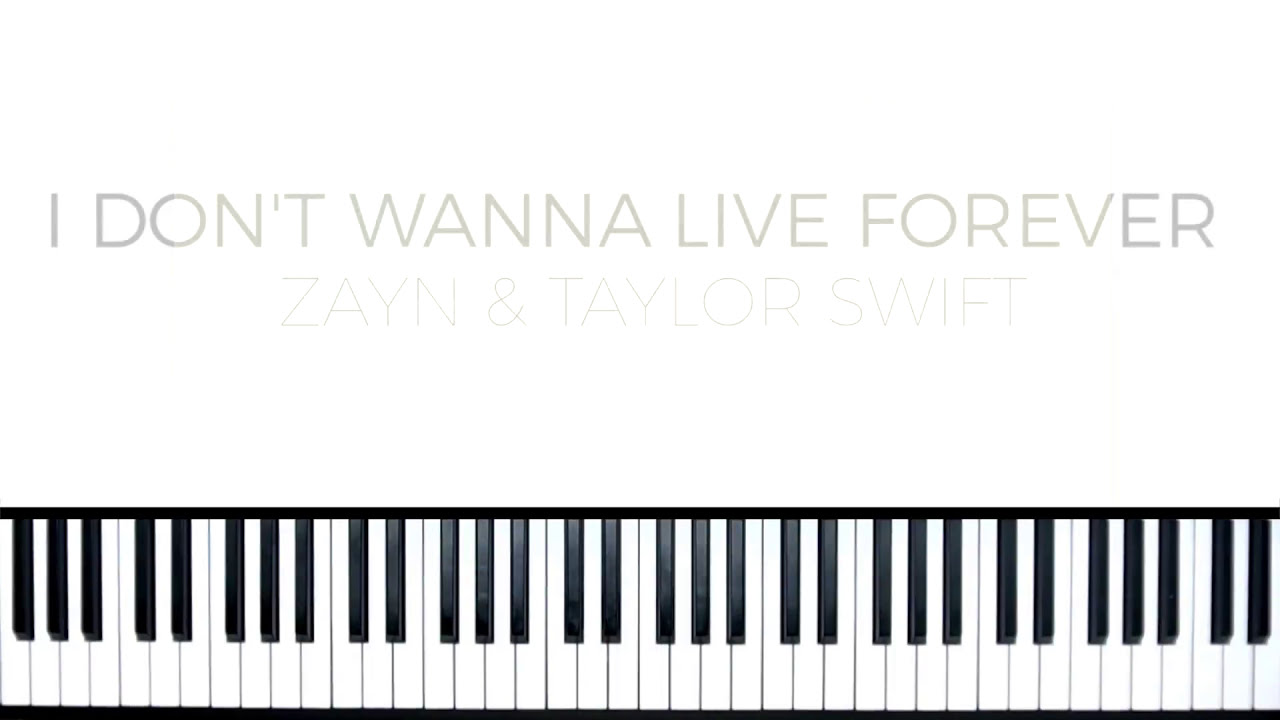The image features a piano keyboard stretching horizontally across the bottom, composed of black and white keys. The keyboard section only displays a portion of keys, starting with an F key and ending with an E key, spanning over five octaves. Above the keyboard, the background is completely white, giving a clean and uncluttered appearance. Centered at the top of the image, there is text in a gray color. The larger, bold, and easily readable line reads "I DON'T WANT TO LIVE FOREVER." Directly beneath it in a smaller, thinner font, also in gray, are the names "ZAYN & TAYLOR SWIFT," with 'Zayn' spelled with a 'Y' and using an ampersand. The overall layout is rectangular, ensuring that the elements are well-spaced and the text is highly legible.